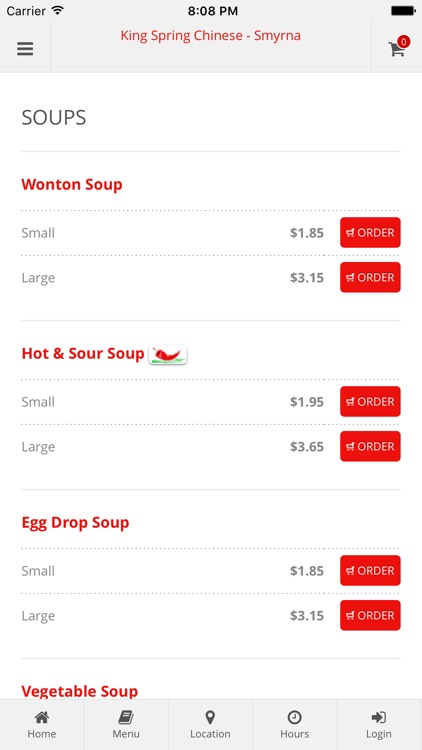The image is a screenshot taken from a cell phone, displaying an online menu for a Chinese restaurant named "King Spring Chinese" located in Smyrna. 

In the top left corner of the screen, it shows the word "carrier," a Wi-Fi signal icon, the time "8:08 PM," and a fully charged black battery icon. 

Beneath this, there are three horizontal black lines representing a menu icon. In the center of the screen, the restaurant name "King Spring Chinese" is in bold red text, followed by "SMYRNA." To the right of this, there is a shopping cart icon with a red "0" indicating that nothing has been added to the cart.

As you scroll down, you enter the "Soups" section. A faint green line separates this section from the title. Underneath, in red text, it lists "Wonton Soup," followed by a faint gray divider line. Below this, the options for "Small" and "Large" are listed. The small wonton soup costs $1.85 and can be added to the order using a grocery cart icon with the word "Order" inside a red rectangle. The large wonton soup costs $3.15 and can also be added in the same manner.

Further down the screen, additional soup options are categorized: "Hot and Sour Soup," "Egg Drop Soup," and "Vegetable Soup." Each of these soup names is displayed in red text. Both the "Hot and Sour Soup" and "Egg Drop Soup" have small and large size options available, with their respective prices shown in gray text. The "Order" buttons for all the soup options are displayed in red rectangles.